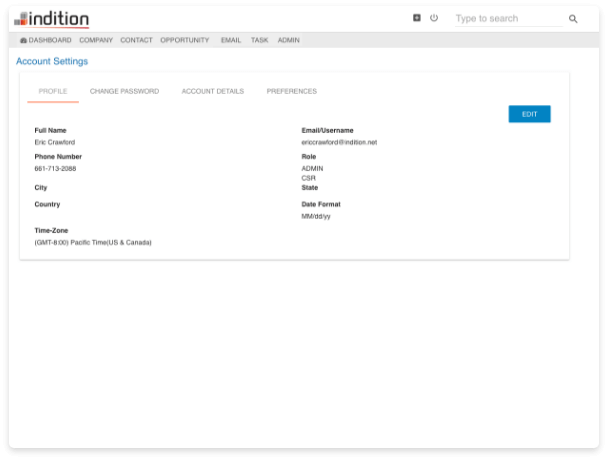A screenshot of the Indition website interface is displayed. The Indition logo, prominently featured in the upper left corner, consists of two squares—an orange square at the bottom overlapped by a gray square, with another gray square adjacent to it. The text “Indition” appears next to the icon, transitioning from a light orange to a darker orange hue from "I" to "N."

Directly below the logo are an on/off button, an indistinct button that is too blurry to identify, and a search bar with a magnifying glass icon.

A vertical menu situated on the left side of the interface lists the following options: Dashboard, Company, Contact, Opportunity, Mail, Task, and Admin. The currently selected Dashboard menu option is denoted with a house icon next to it. The menu is set against a gray rectangular background.

Below the vertical menu, there is a box outlined in gray with a white background that reads "Account Settings" in aqua blue text. The box has tabs labeled Profile, Change Password, Account Details, and Preferences, with the Profile tab currently selected.

The Profile section details the user's information:
- Full Name: Eric Crawford
- Phone Number: 661-713-2088
- City: (blank)
- Country: (blank)
- Time Zone: GMT -8, Pacific Time, US and Canada
- Email/Username: eric.crawford@edison.net
- Role: Admin CSR
- State: (blank)
- Date Format: MM/DD/YY

To the right of these details is an Edit button colored blue with white text. The rest of the interface consists of white space.